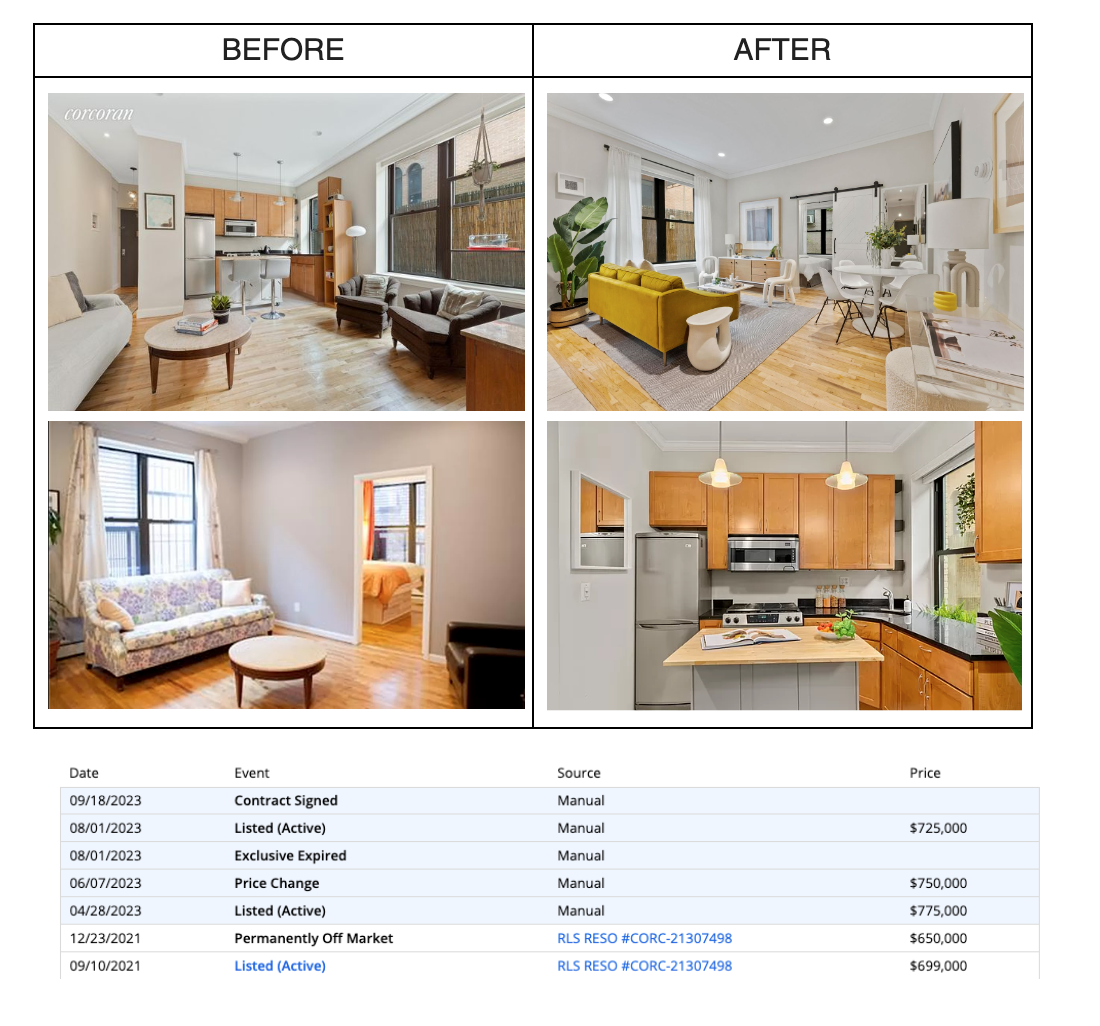Screenshot Description: Home Renovation Before and After Comparison

This image showcases a side-by-side comparison of a home renovation with "Before" and "After" columns at the top. 

**Top Row:**
- **Before:** The first image displays an open-plan living room and kitchen area. The living room features white and gray furniture, including a round coffee table. The kitchen in the background is compact, with stainless steel appliances and wooden cabinets. A window to the right reveals a view of a brown wooden fence.
- **After:** The same living room and kitchen area are shown, now redecorated. The contemporary look includes a new yellow couch and updated furnishings. In the back of the room, a sliding barn door has been added on a track, enhancing the modern decor.

**Middle Row:**
- **Before:** The second image presents an outdated couch with a purple floral pattern. Through a doorway in the background, part of a bed in another room is just visible.
- **After:** The updated image now highlights the kitchen area, where an island has been installed. The original cabinetry and stainless steel appliances remain, but the new counter is dark and shiny, adding a modern touch.

**Bottom Section:**
- The lower part of the screenshot lists chronological data about the property's status and pricing changes:
  - **9-18-2023:** Contract signed, manual, $725,000
  - **8-1-2023:** Listed active, manual, $725,000
  - **8-1-2023:** Exclusive expired, manual, $750,000
  - **6-7-2023:** Price change, manual, $750,000
  - **4-28-2023:** Listed active, manual, $775,000
  - **12-23-2021:** Permanently off-market, RLS, RESO, #CORC-21307498, $650,000
  - **9-10-2021:** Listed active, RLS, RESO, #CORC-21307498, $699,000